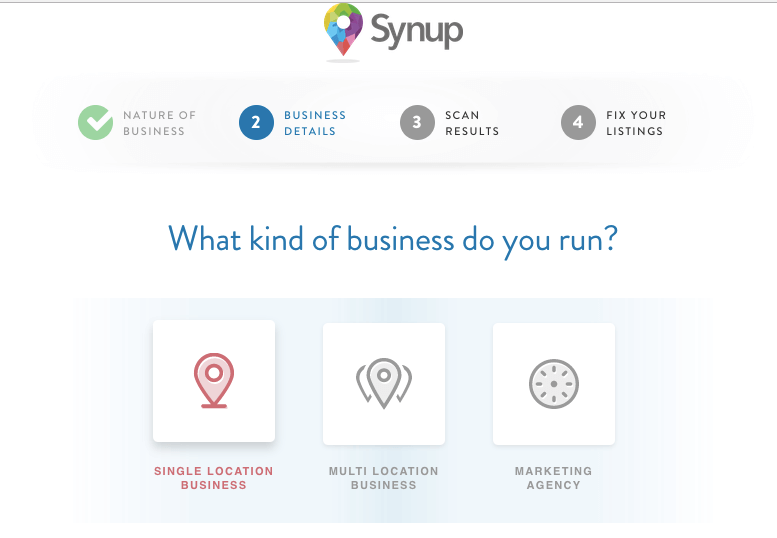The image features a top section with a light gray horizontal line. Just below this line is a location pin that vertically transitions through every color of the rainbow: it begins with red at the base, followed by blue, pink, purple, orange, yellow, and ends with green at the top. To the right of this colorful pin, the word "Synup" is written in black, with each letter in uppercase. Underneath the pin, another small horizontal gray line appears, followed by a sequence of elements.

Directly below this, there is a gray rectangular box. Inside this box, from left to right, are:
1. A green circle with a checkmark, accompanied by the text "The Nature of Business."
2. A blue circle with the number "2" inside, adjacent to the text "Business Details."
3. A gray circle with the number "3" inside, next to the text "Scan Results."
4. Another gray circle containing the number "4," alongside the text "Fix Your Listings."

Below this box, a blue text caption reads, "What kind of business do you run?" Beneath this caption is a larger blue rectangular box housing three white squares. 

The leftmost square contains a red location pin icon, underlined by the red capital text "Single Location Business."